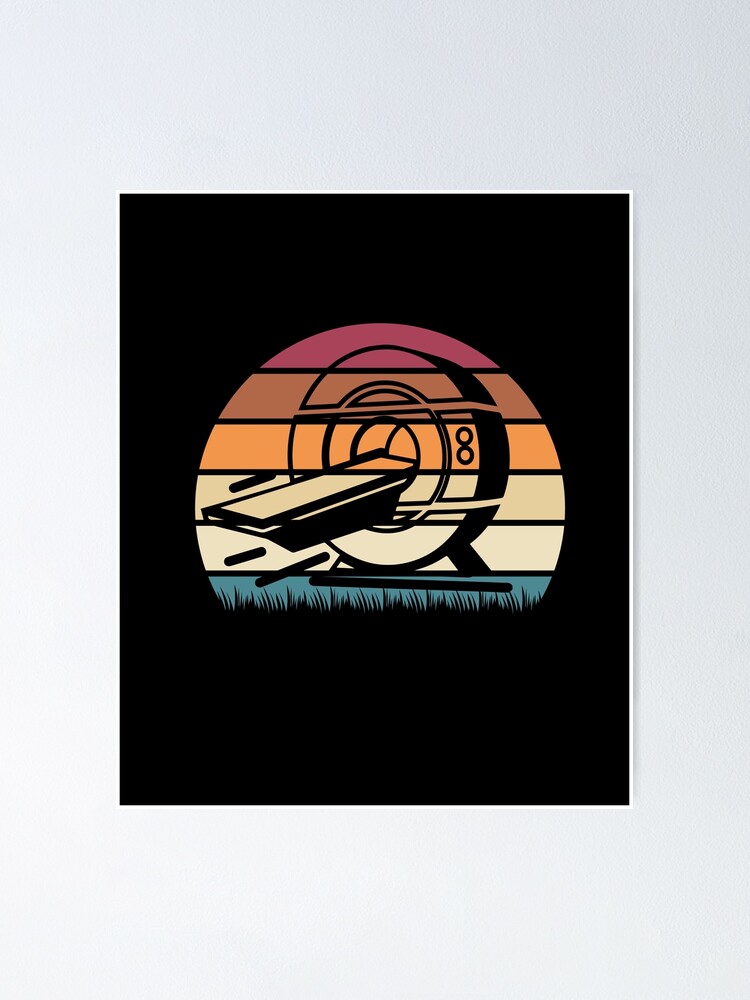The image features a stylized, abstract poster centrally aligned on a light gray wall. The poster itself has a solid black background bordered by a thin white line. Dominated by a large, partial circular design, the top and sides of this circle are visible, while the bottom portion is obscured by black silhouettes of grass. Extending from the center of the circle is a plank-like element, giving the impression of a platform extending outward. On the right side of the circle, two smaller circles form a figure-eight.

Within the circle, the design comprises horizontal bands in a sequence of colors. From top to bottom, the shades progress from fuchsia (or pinkish-purple), brown, orange, to tan and beige. These colored bands are separated by horizontal black lines. The bottom section of the circle features blue bands, above which the silhouettes of grass are apparent. The overall appearance is reminiscent of abstract art, blending geometric elements with a gradient of warm, earthy tones, aurally representing a blend of natural and constructed forms.